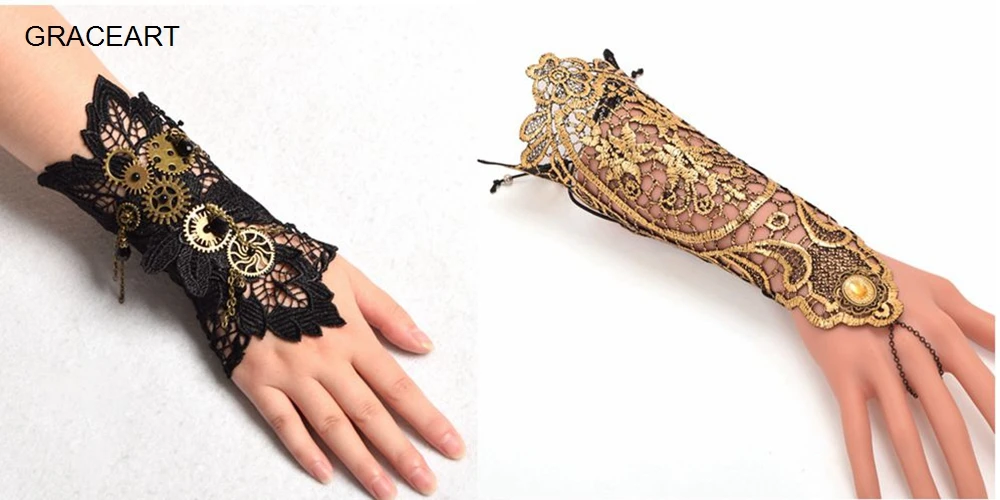The image advertisement, labeled "GRACE ART" in the upper corner, showcases two distinct decorative wrist cuffs, each featured in separate photographs. Both images depict an arm extending from the upper corner, fingers pointing towards the bottom right. The left photograph illustrates a real hand, adorned with a black lace cuff reminiscent of steampunk style. This cuff, extending from just below the knuckles to about mid-forearm, is embellished with various brass gears aligned down the wrist and has a leaf-like lace design. The background here is textured white, accentuating the delicacy and contrast of the black lace against the pale skin.

In contrast, the right photograph displays a mannequin hand against a solid white background, wearing a lacy gold cuff. This cuff, mixed with hints of black lace, features a chain that wraps around the middle finger, topped by a jewel resembling topaz or gold. This longer cuff extends from the knuckles to nearly the elbow, showcasing a more intricate and pointed design. Both images harmoniously highlight the elegance and craftsmanship of the fingerless gloves, emphasizing the intricate lacework and ornamental details.